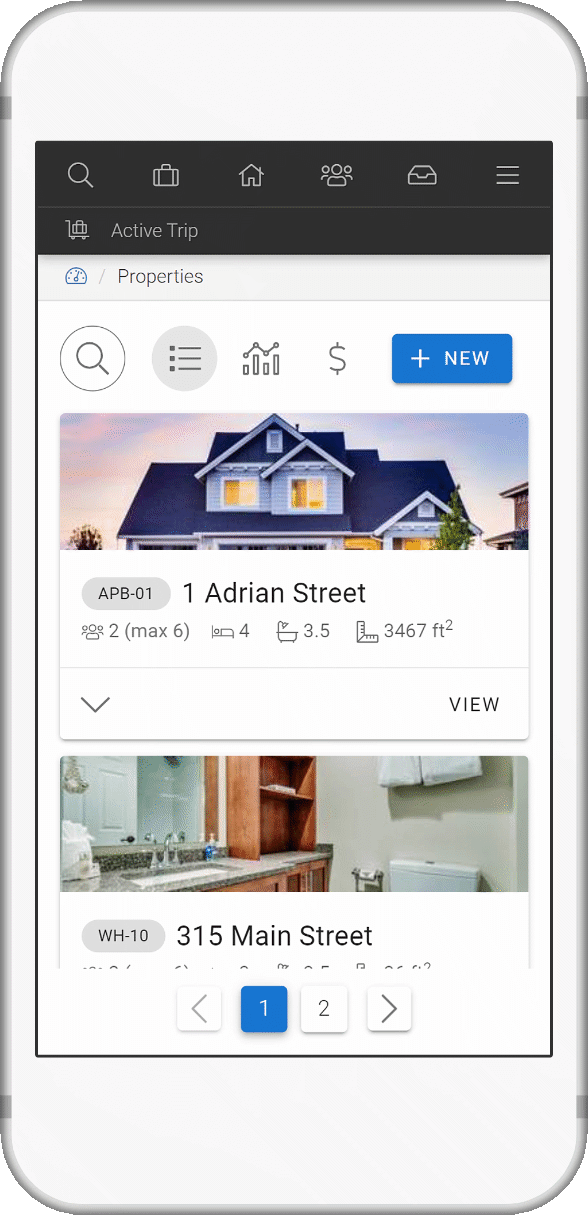The image depicts an iPhone with a classic Apple design, featuring a white top and bottom, a silver border, and a black border at the top of the screen. Within the black border, there are several icons: a white magnifying glass, a suitcase, a phone or house symbol, a group of three people illustrated as small heads with shoulders, a tray, and three horizontal lines stacked with small spaces in between.

Further down the screen, there is an icon resembling a dolly or push cart with a suitcase on it and the text "Active Trip," with "A" and "T" capitalized. Below this section, there's a white banner displaying the word "Properties". 

The main content area of the screen, which has a white background, contains two circular icons. The first circle has a white background with a magnifying glass icon inside it. The second, a gray circle, features three horizontal lines with dots in front of them. Next to these is a dollar sign icon and a blue button labeled "Plus New."

Beneath these elements, there are textual entries indicating property addresses. One entry shows a house labeled "1 Adrian Street," and another shows a bathroom labeled "315 Main Street."